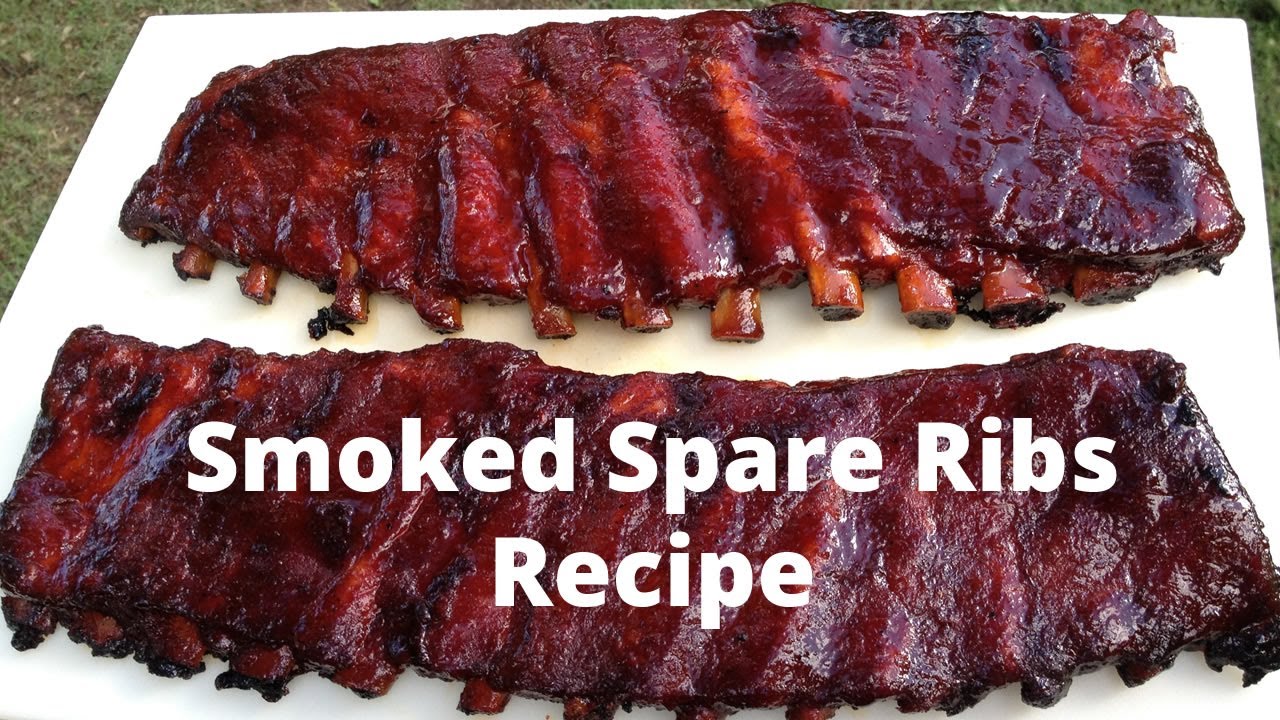The image captures two racks of succulent spare ribs positioned on a white table against an outdoor backdrop with hints of grassy ground at the edges. The top rack, smaller in size, boasts a glossy red barbecue glaze with bones protruding, signifying a well-cooked masterpiece. The bottom rack is larger, featuring a mix of charred patches and the same enticing glaze, creating a visually appealing contrast of textures and colors. Both racks glisten under what seems to be a slow roasting process that locked in the flavors. Dominating the scene in large white text across the bottom rack are the words "Smoked Spare Ribs Recipe," suggesting this could be a promotional image or a still from a culinary video or website.